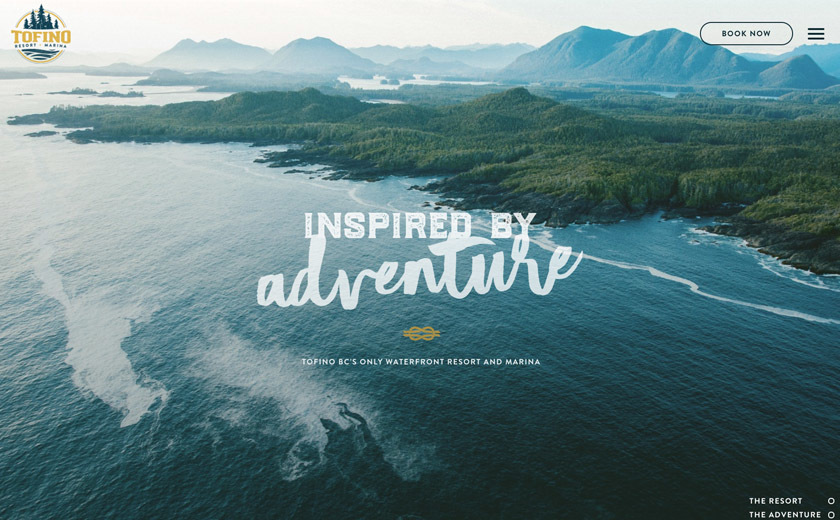This image depicts the front page of a website for Tofino Resort and Marina. In the background, a serene and foggy landscape features majestic mountains covered in lush greenery, with the lower part of the image showcasing a dark, slightly wavy ocean. Centered across the image is white text that reads "Inspired by Adventure" with "Tofino BC's only waterfront resort and marina" underneath in smaller font. In the top left corner, a round logo with trees and the text "Tofino Resort Marina" is visible. The top right corner contains a "Book Now" button alongside a small sandwich menu icon with three horizontal lines. Near the bottom of the image, additional text states "the resort" and "the adventure," emphasizing the theme of exploration and natural beauty.